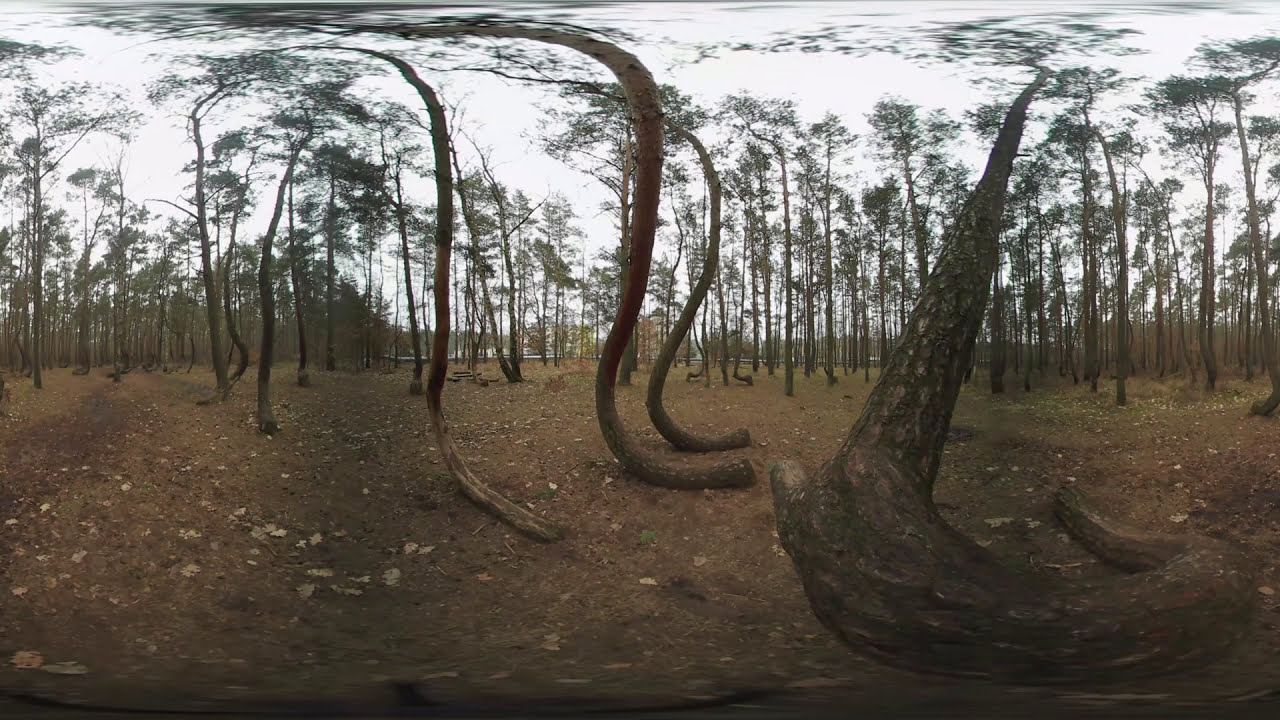This photograph captures a forest scene with a unique perspective that distorts the natural elements. The ground is predominantly brown, with patches of grass and scattered rocks. Dominating the landscape are numerous tree trunks, some of which exhibit a striking backwards S shape, giving them a snake-like appearance. This unusual distortion is likely due to the use of a 360-degree or panoramic lens, which warps the usual straight lines of the trees, especially those in the foreground. The trees further in the distance appear straighter and more traditional in form. Sparse foliage decorates the upper parts of the trees, with leaves appearing somewhat blurred and misaligned, enhancing the surreal quality of the image. The sky behind the forest canopy is a hazy white, adding a stark contrast to the earthy tones below and emphasizing the ethereal, almost otherworldly atmosphere of the scene.